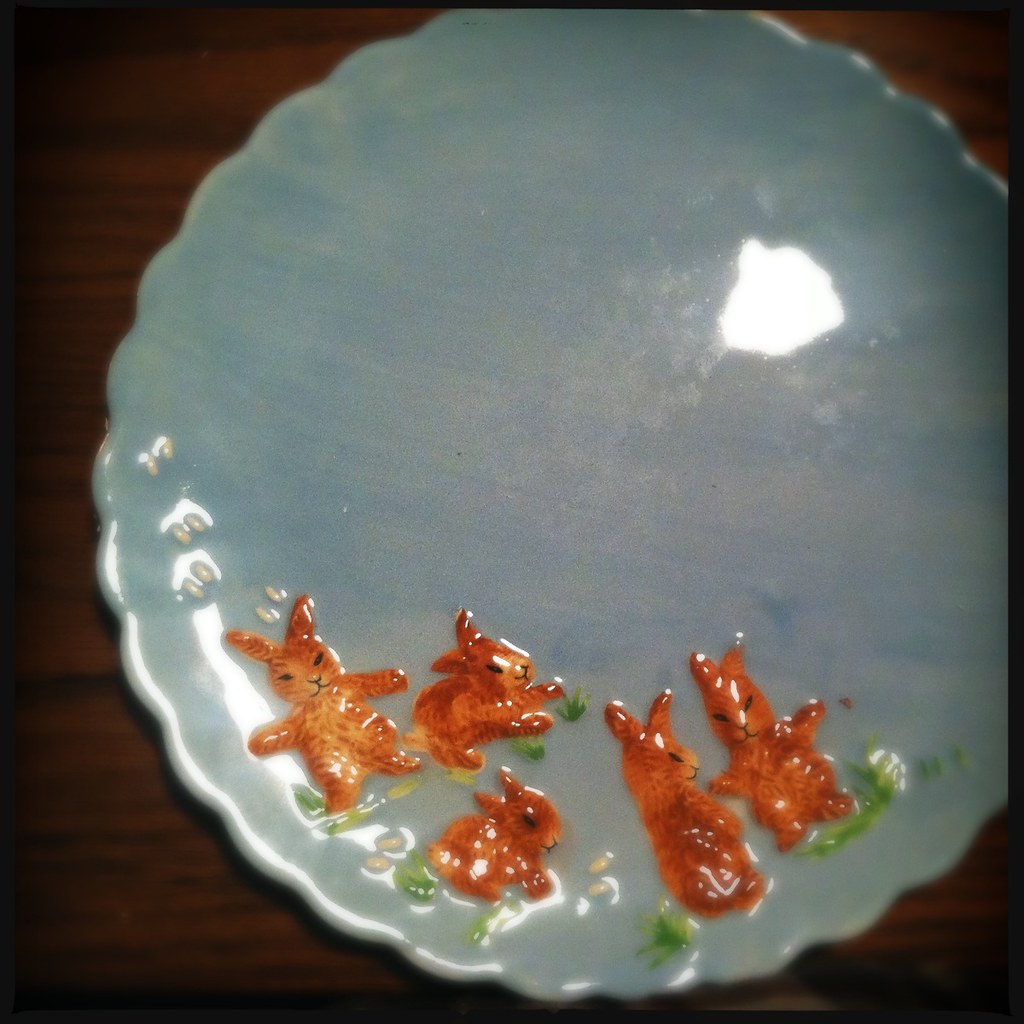This close-up color photograph captures a beautifully detailed ceramic plate resting on a dark brown wooden table, likely indoors. The plate, positioned centrally in the image, features a striking blue surface punctuated by light stripes of yellow and a scalloped, sinusoidal ridge pattern on its edge. Prominently displayed on the plate are five rust-colored bunny rabbits depicted in various poses: two are hopping, while the other three stand on their hind legs. The scene is enhanced by small white footprints and tufts of grass surrounding the bunnies. The reflection of the camera's flash can be seen on the plate's surface, adding an element of realism to this intricately designed, high-quality piece.